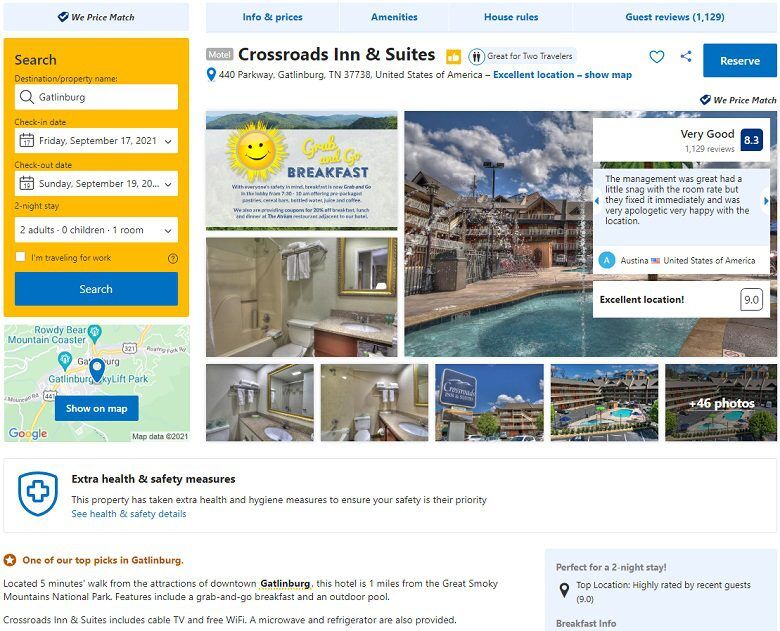A webpage interface for a hotel booking site is described in detail. At the top of the page, several clickable buttons are arranged within a light blue bezel, featuring dark blue text labels: "Info & Prices," "Amenities," "House Rules," and "Guest Reviews (1127)." Below this section, against a white background on the left side, is a gray rectangle with white text reading "Motel." Adjacent to this, "Crossroads Inn & Suites" is prominently displayed in bold black text. An up arrow is positioned beneath this, followed by a dark blue pin icon indicating the address: "440 Parkway, Gatlinburg, Tennessee, 37738, United States of America" with the location spelled out as "G-A-T-L-I-N-B-U-R-G." To the right, a blue hyperlinked text states "Excellent location – show map."

On the far right, icons for a heart and share symbol appear next to a dark blue rectangle with white text reading "Reserve." On the left, within a light blue bezel, there's a dark blue tag next to "We Price Match" in black text. Below this section, an orange rectangle contains "Search" in black text. 

Further down, the page displays a search area with "Destination/Property Name" and an input field containing "Gatlinburg" with a magnifying glass icon. Underneath, it details the "Check-in Date" with a calendar icon, set to "Friday, September 17th, 2021," the "Check-out Date" with another calendar icon, set to "Sunday, September 19th," though the year is truncated. Just above the final dropdown menu, "Two Night Stay" is logged with "2 adults, 0 children, 1 room."

A white square labeled "I'm traveling for work" with a black circle enclosing a question mark on an orange background appears but is unchecked. Below this, another dark blue rectangle marks the central "Search" button. Lastly, a small map of Gatlinburg Lift Park showcases a dark blue rectangle reading "Show on Map," followed by images of the hotel’s interior, exterior, and large pool area.